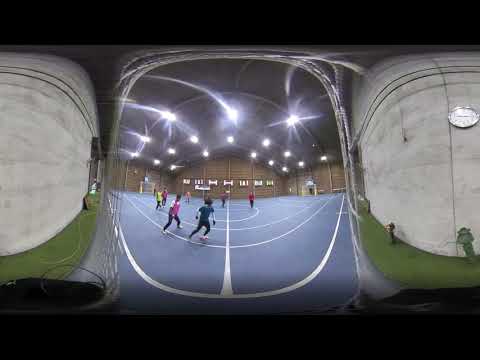The image depicts an indoor sporting activity taking place on a blue field marked with white stripes. The spacious gymnasium features bright overhead lighting, illuminating the scene vividly. The field hosts two teams, with around nine or ten players in total, including goalies on either side. The athletes, dressed in long-sleeved shirts and pants, are scattered around the field, seemingly engaged in a dynamic game. The building's walls are brown, reminiscent of wooden beams or a log cabin, and the ceiling is dark gray. Windows line the back wall, interspersed with a few doors. Several children, both boys and girls, are visible, some running and others walking or playing. In the foreground, a boy in a blue shirt and black pants is running, with a girl in a pink and white shirt and black pants close behind him.